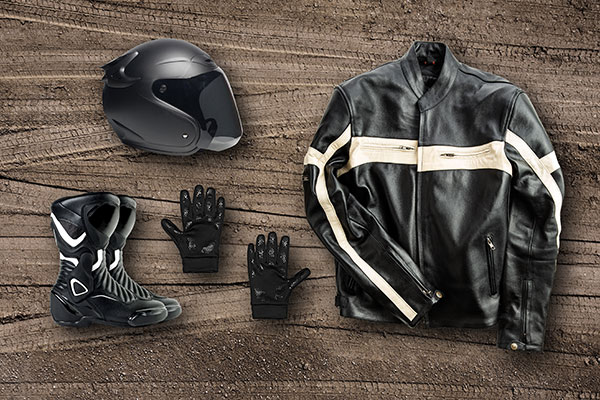The image depicts an array of black motorcycle gear arranged systematically on a treaded, textured surface that appears grayish-brown, resembling dirt with tire tracks. Positioned on the right side is a black leather motorcycle jacket adorned with horizontal white stripes on the sleeves and chest, complete with a horizontal zipper pocket. To the left of the jacket, in the upper section of the image, is a black motorcycle helmet with a dark visor oriented to the right. Directly below the helmet, near the left side, are a pair of black leather motorcycle boots with white accents, both facing to the right. Adjacent to the boots, to the right, lies a pair of black leather motorcycle gloves arranged with the left hand glove on the left and the right hand glove on the right. The camera captures a top-down view, showcasing these meticulously placed items against the distinctive patterned backdrop.